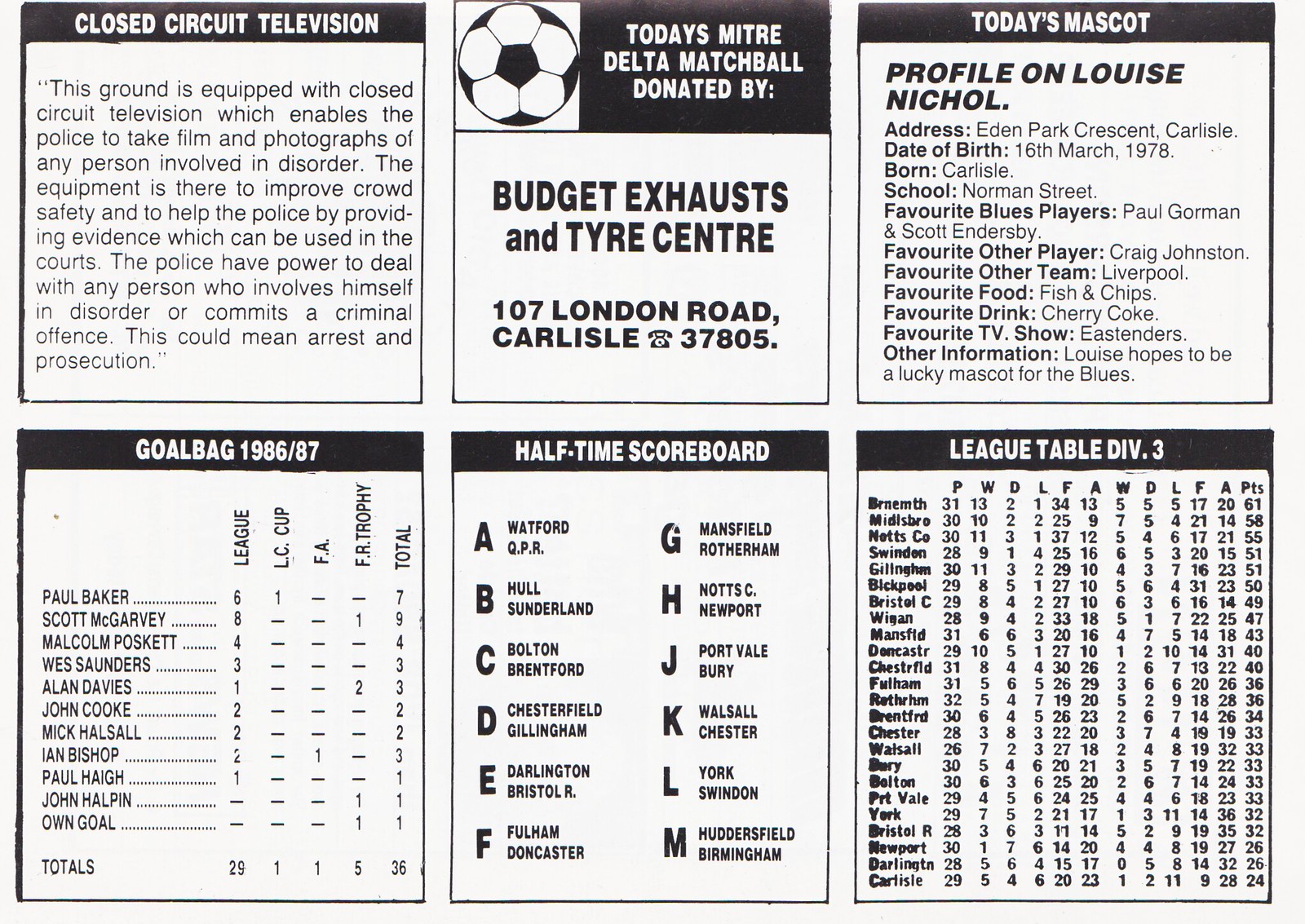This black-and-white program page, likely from a sports magazine or event program, is filled with detailed information across various sections. At the top left, there's an article titled "Closed Circuit Television," explaining the ground's surveillance capabilities for monitoring and recording any disorderly conduct. In the top middle, an advertisement highlights "Today's MITRE Delta Match Ball Donated By Budget Exhaust and Tire Center," accompanied by a soccer ball image. The top right section features "Today's Mascot Profile" of Louise Nicole, including personal details such as date of birth and the school attended. 

The bottom half of the page is dedicated to team statistics. On the bottom left, the "Goal Bag 1986-87" section lists player goal statistics. The central bottom section, marked "Halftime Scoreboard," displays updates from various teams. Finally, on the bottom right, a "League Table Division III" scorecard provides league standings and related statistics. The entire layout is presented in a clean, black-and-white format, structured into six segments with an emphasis on informative content and team data.